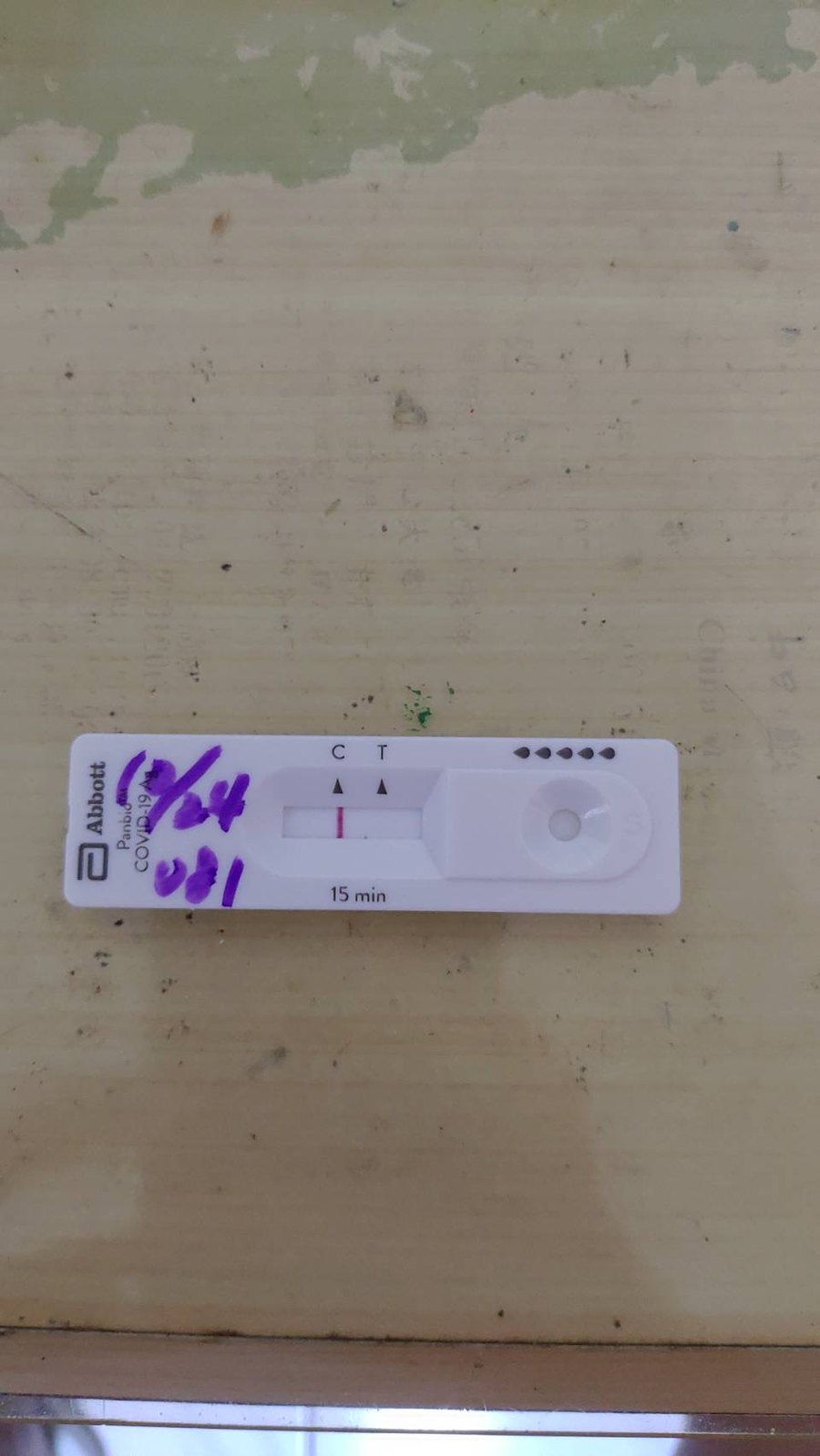The image depicts a light-colored wooden table with a noticeable splotch of green paint at the top. Centrally positioned on the table is a horizontal Abbott PanBio trademarked COVID-19 antigen test. The test features a white rectangular section above a window, marked with the letters "C" and "T." A prominent bright pink line is visible directly under the "C," indicating a negative result. Below the window, the test reads "15 min." In the bottom right corner, there are five small black teardrop shapes. Along the left side of the test, "10/24" is written in purple marker, with an additional, somewhat illegible note below it, possibly reading "081." The overall image has a vertical orientation, being much taller than it is wide.